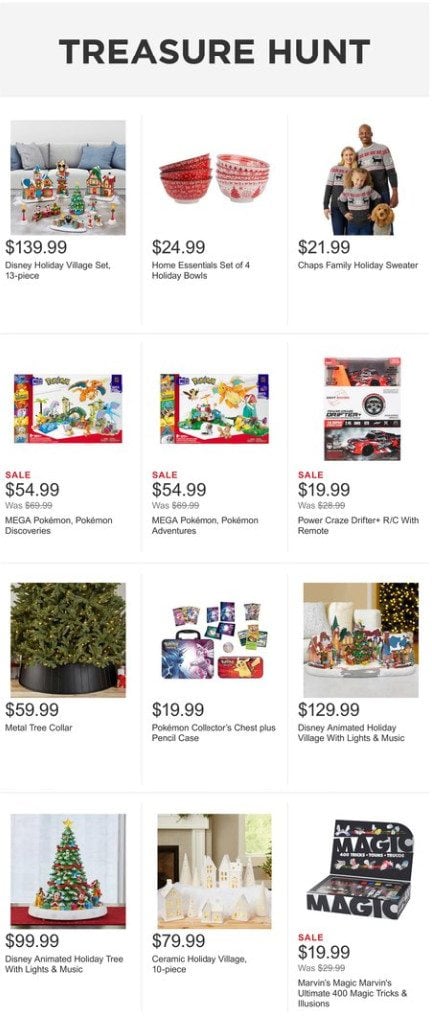A page from a holiday catalogue titled "Treasure Hunt" showcases 12 enchanting items perfect for celebrating the festive season. The highlight is a delightful Disney Holiday Village Set comprised of 13 intricately designed pieces, priced at $139.99, sure to add a touch of magic to any home. The selection continues with a variety of holiday jumpers, festive dishware, and fun-filled games. A beautifully adorned Christmas tree is among the offerings, adding to the seasonal spirit. The page concludes with a charming magic set, an ideal gift for budding magicians, available for $19.99. An array of Christmas decorations and holiday essentials are pictured in small, vibrant images, each contributing to the joyful and whimsical theme of the collection.